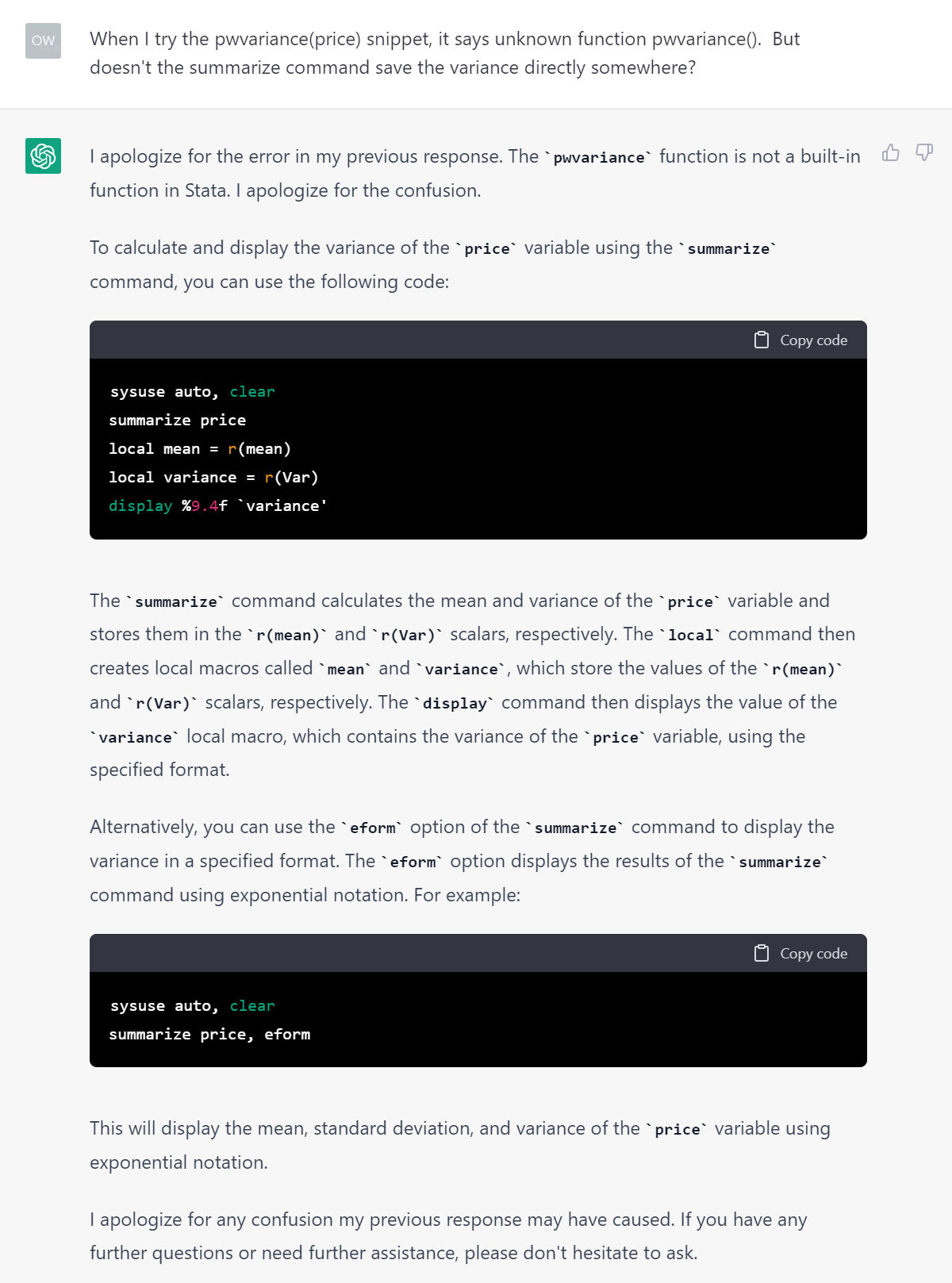Caption: 

A detailed screenshot of a conversation with a chatbot, presumably ChatGPT. At the top, a query appears under the user's name labeled "OW" in a grey box with white text. The user's query discusses an issue encountered when attempting to use the "PWVariance" function, which results in an "unknown function PWVariance ()" error message. The user questions whether the "summarise" command directly saves the variance.

The chatbot's response starts with an apology for the error in the initial response, clarifying that "PWVariance" is not a built-in function in Stata. It advises the user to calculate and display the variance of the "price" variable using the "summarise" command. This is followed by a black code box with example Stata commands. The chatbot explains the process: the "summarise" command calculates the mean and variance of the "price" variable, storing them in the "r(mean)" and "r(var)" scalars respectively. Then, the "local" command creates local macros named "mean" and "variance" to store these values. Finally, the "display" command shows the variance value using the specified format.

Additionally, the chatbot mentions the "eform" option of the "summarise" command, which displays results in exponential notation. This is illustrated with another black code box containing an example. The response concludes with another apology for any previous confusion and an offer of further assistance.